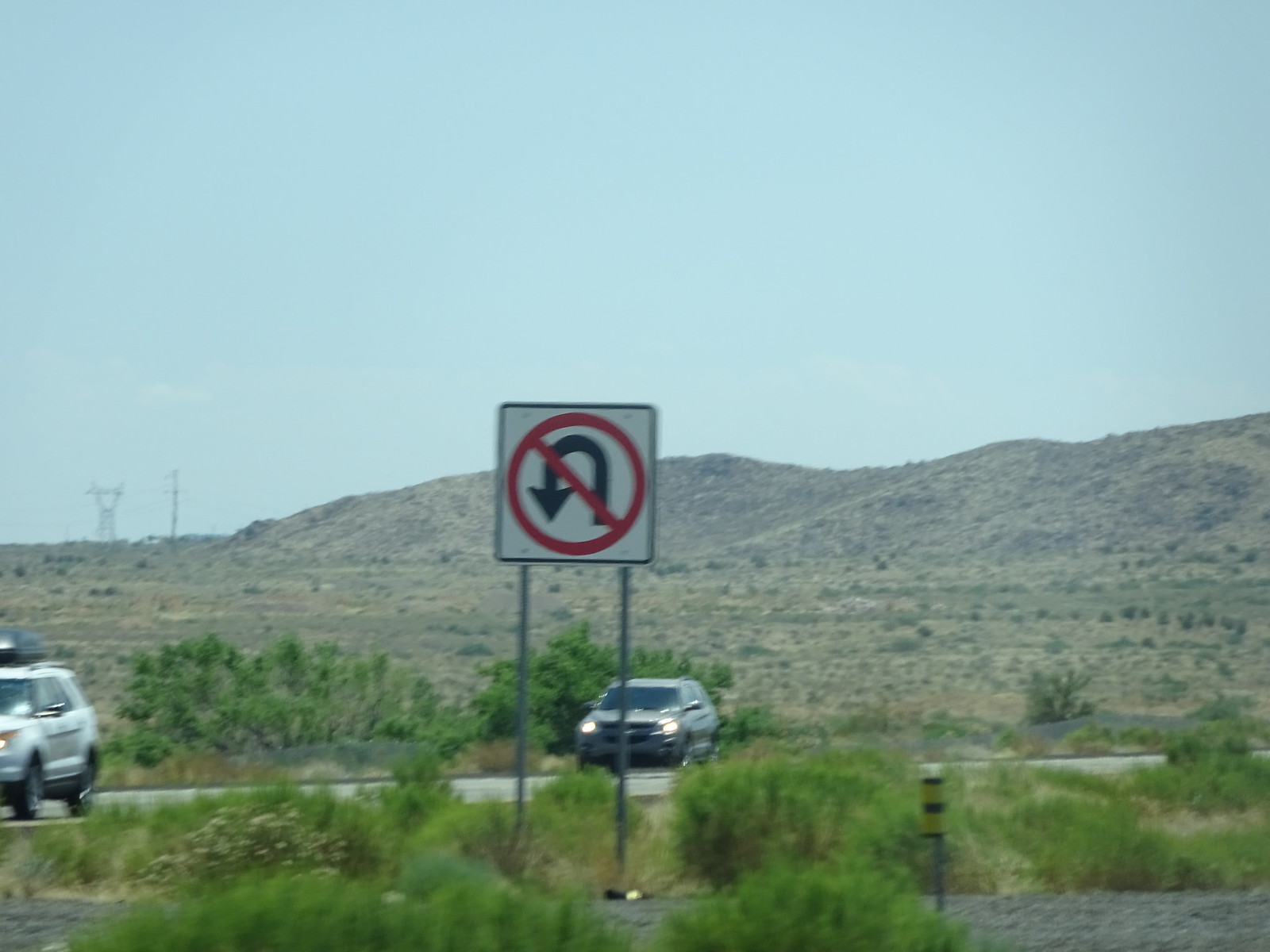In the midst of an expansive, deserted landscape, a lone road stretches into the horizon. Tall poles adorned with yellow and black caution tape line the roadside, standing as silent sentinels. Short, green plants dot the gravel-strewn ground, adding a touch of life to the barren surroundings. Two cars make their way down the road, seemingly tiny against the vast backdrop. A prominent road sign, supported by two silver posts, stands tall. The sign, stark white with a bold red circle and a curved arrow crossed out by a red line, clearly indicates that U-turns are prohibited. In the distance, majestic mountains rise against the blue sky, while towering power lines loom on the far horizon, completing this scene of isolation and rugged beauty.